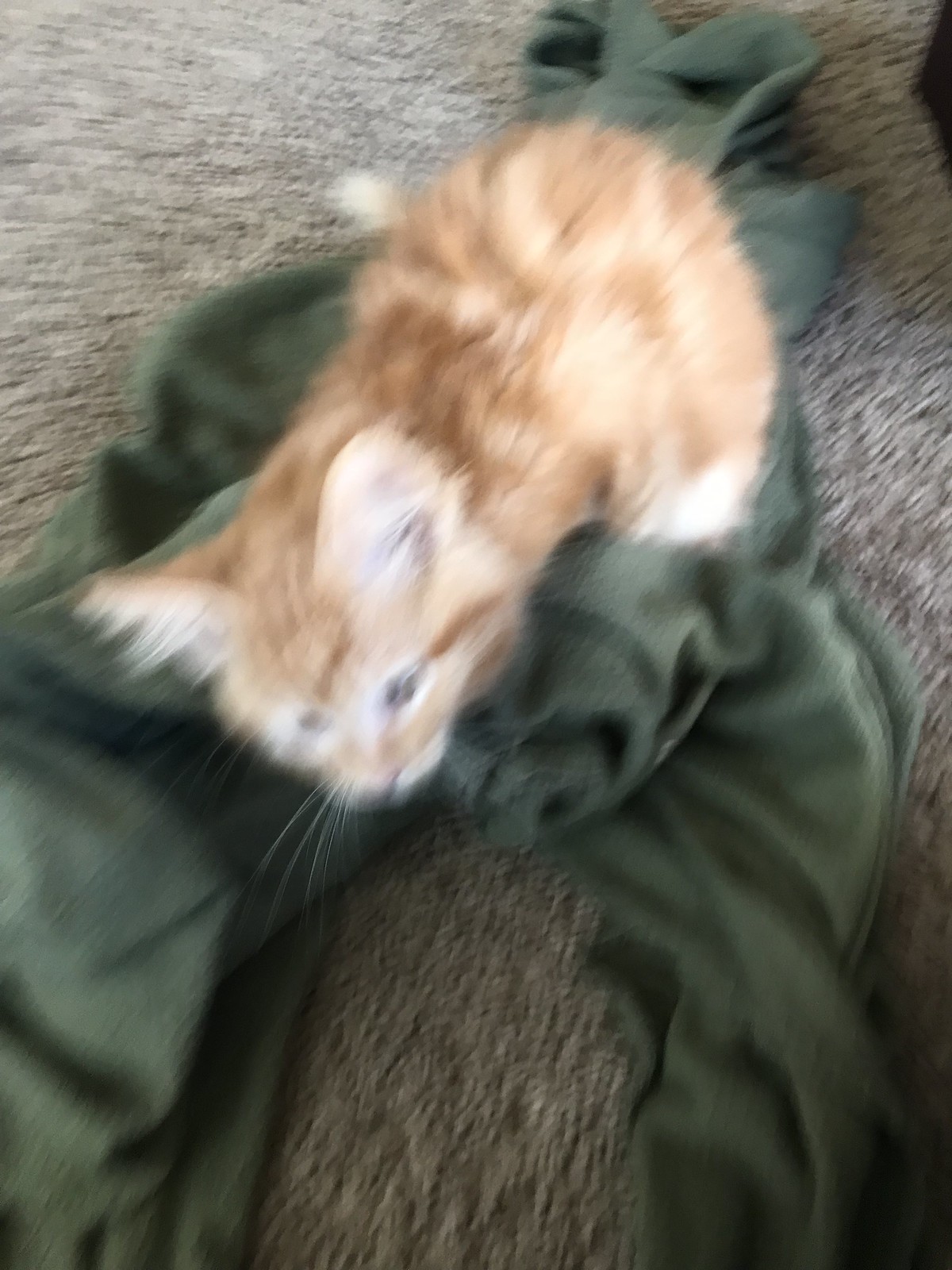The image is a slightly blurred, indoor color photograph featuring a ginger-colored cat as the main subject. The cat is sitting on a dark, muddy green article of clothing, likely a pair of sweatpants, which is strewn across a short-pile brown carpet. The photograph is taken from a 45-degree downward angle, allowing a view of the top of the cat's head and the inside of its ears, which point upwards. The cat appears alert, with its eyes open and a mix of orange and white fur, including white patches in its ears, around its eyes, and along the lower snout. The sweatpants have a distinctive ribbed waistband, adding to their identification. The carpet beneath features varying shades of brown with lighter, almost off-white tones interspersed throughout, creating a textured appearance.